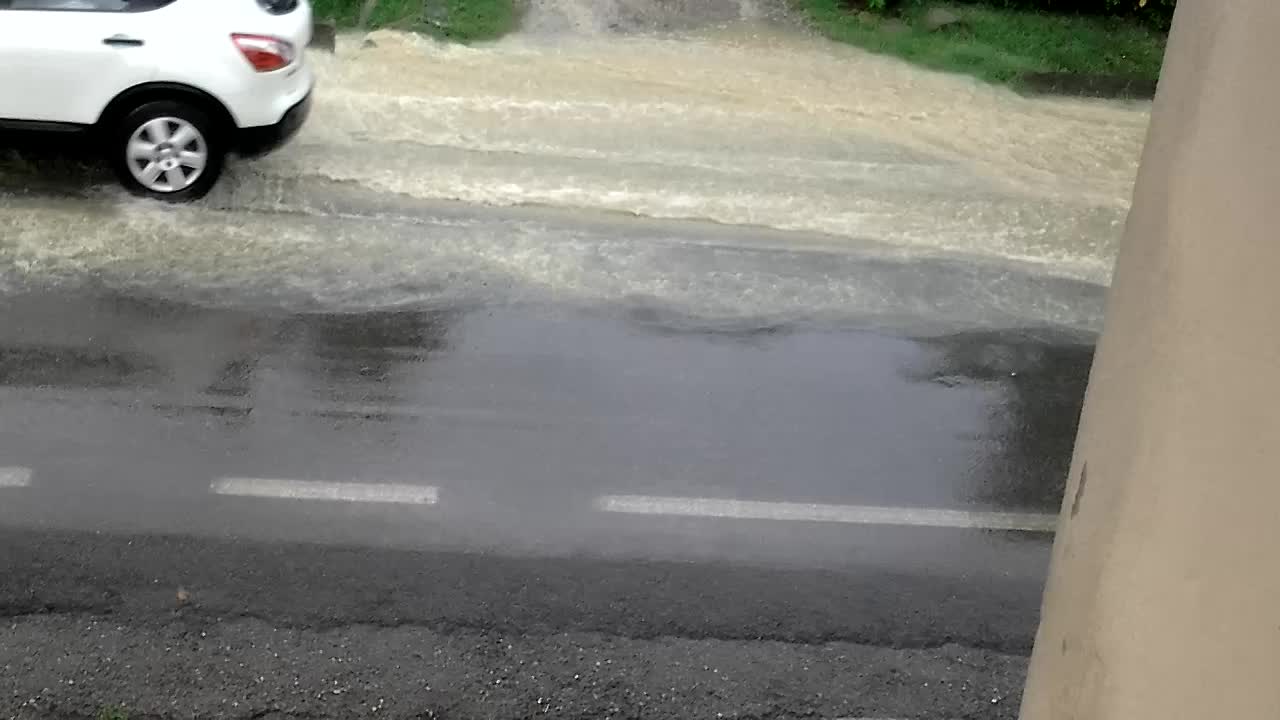The photograph depicts a rainy street scene from an elevated perspective, potentially taken by someone standing inside an overhang or on a staircase. The lower third of the image shows a detailed view of the road, beginning with gravel near the bottom, leading to a strip of darker asphalt, and then the main road featuring white, spaced lines running horizontally. The road surface is glossy and reflective, indicating recent rainfall. A large pool of dirty gray water partially floods the upper portion of the street, suggesting a clogged drain.

A white SUV is navigating through the water in the upper left corner of the image. This vehicle’s aluminum hubcaps and dark black tires are visible, along with the back door handle and a small part of the window. Tire tracks mark its path through the shallow flood. There is green grass visible behind the car and extending to the right side of the photo. On the right-hand side of the frame, a tan concrete wall suggests the photograph might be taken from a stairway or window. This wall protrudes outward, reinforcing the idea of a structure's staircase being in the frame.

The overall scene is framed by urban elements, emphasizing the flooded road as the central focus of the photograph.